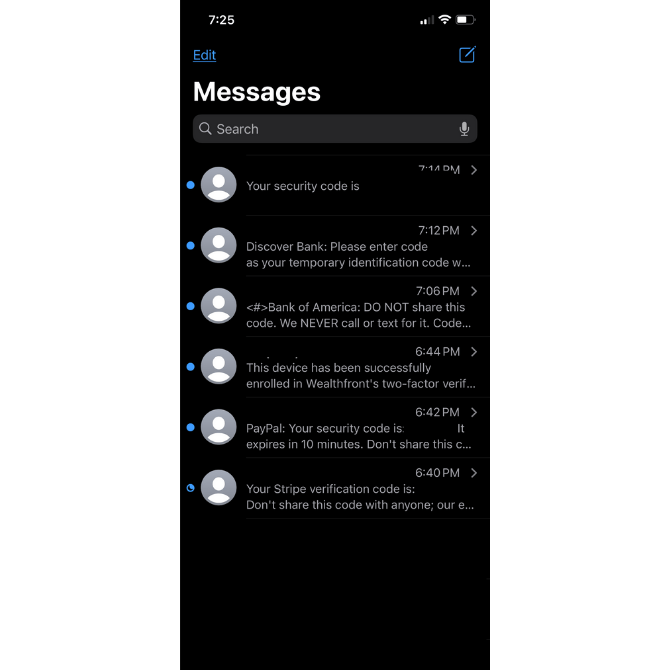The screenshot depicts a smartphone screen displaying the time as 7:25, with two signal bars, an active Wi-Fi connection, and approximately three-quarters battery life remaining. At the top right, there’s an "edit" hyperlink accompanied by a pencil icon and another pencil-and-paper icon.

The main heading on the screen is "Messages" written in large, bold white letters. Below this heading, there is a gray search box featuring a magnifying glass symbol and a microphone icon. 

Further down, each line shows a blue circle on the left, representing the notification indicator for unread messages. To the right of these circles are generic profile pictures, each consisting of a simple circle head on a gray background. On the far right of each line is the timestamp and a greater-than symbol, signifying that these are incoming messages.

The content of the messages displayed is as follows:
1. The top message reads, "Your security code is"
2. The next message from "Doge Bank" requests, "Please enter code as your temporary identification."
3. The final message from "Bank of America" warns, "Do not share this code; we never call or text for it."